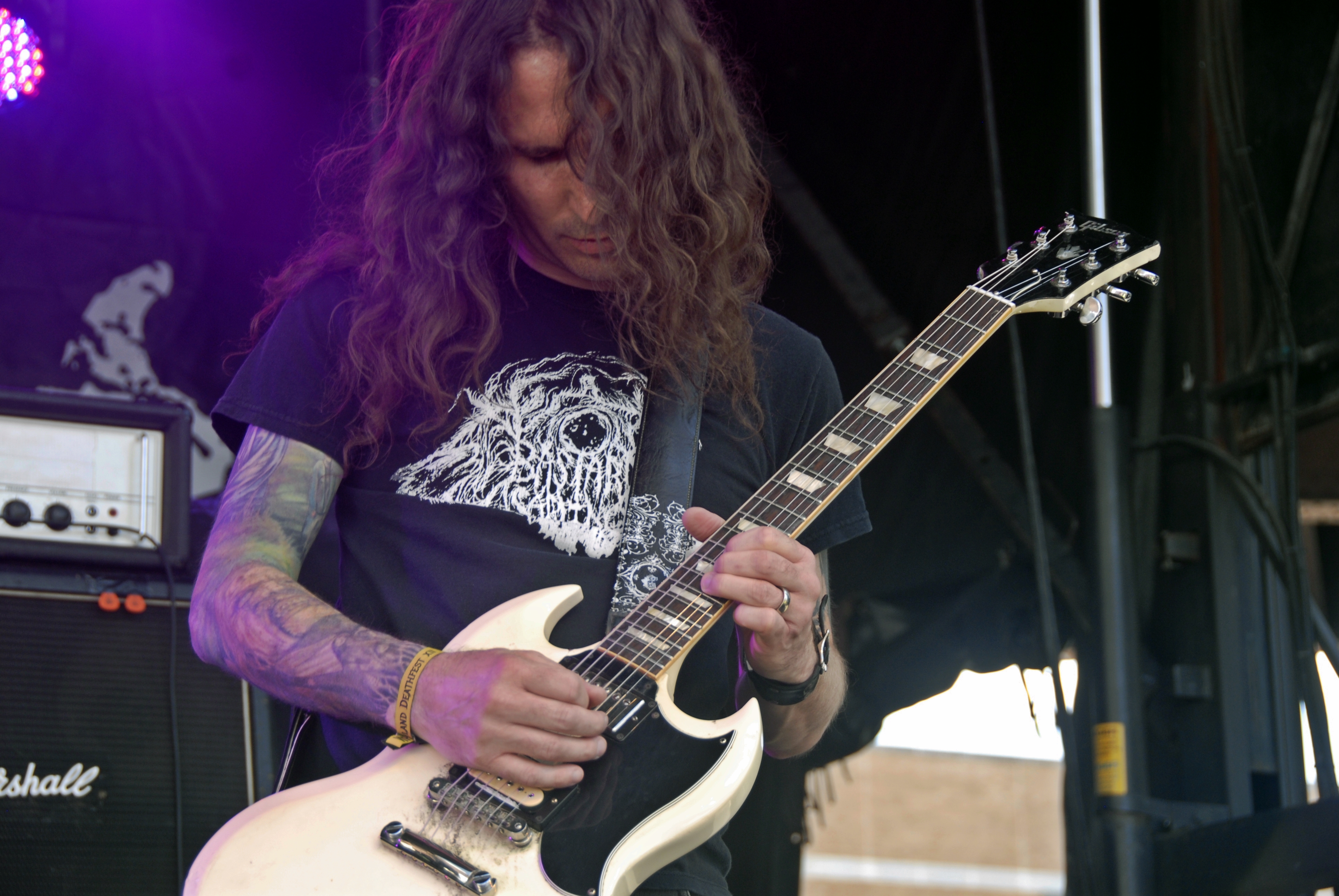The image features a man with long wavy brown hair obscuring his face as he looks down, intently playing an off-white, ivory guitar with black detailing. He is dressed in a black short-sleeved t-shirt adorned with a white pattern resembling an animal's eye. His right arm is fully tattooed and he wears a yellow wristband with the text "DEATH FEST" in black. The background reveals various band equipment, including a microphone stand and audio gear, suggesting a performance setting. A purple curtain and a glimpse of tan flooring can also be seen, along with an outdoor view through a gap, indicating he is performing in a covered area.